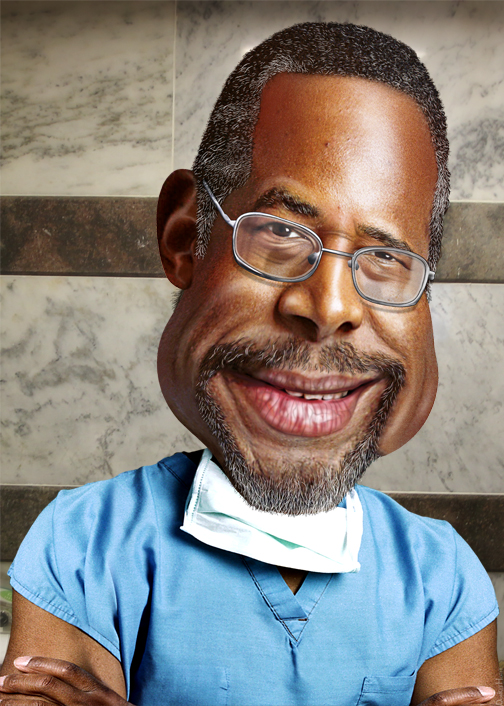This image appears to be a digitally altered or comic-styled portrayal of an African American individual bearing a resemblance to Barack Obama, although it is unclear if it is indeed him. The person in the image is dressed in a blue shirt and situated against a backdrop of marble tiles, indicating an indoor setting. Noteworthy details include the subject's very short hair and exaggerated facial features—specifically, both sides of the face, the lips, and the mouth, which have been distorted for a comical or satirical effect. Additionally, the glasses worn by the individual appear to be AI-generated, further suggesting a digital or artistic manipulation aimed at creating a political or satirical commentary.